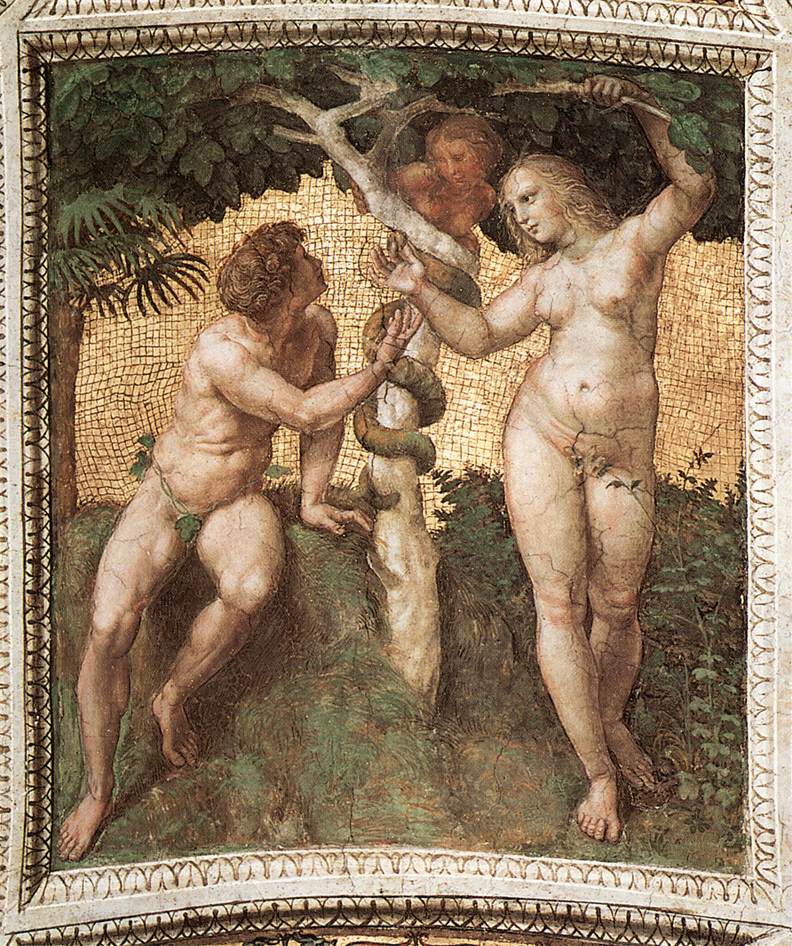This painting is a detailed and realistic depiction of the Garden of Eden, featuring three prominent nude figures. The central figure is a tree with lush green foliage at the top and grass with weeds at its base, all set against a neutral tan background. On the right-hand side stands Eve, a nude woman with wavy blonde hair cascading below her shoulders. She is partially covered by weeds and flowers growing around her body and is gripping the tree branches, her cracked skin adding a layer of texture to her portrayal. 

On the left is Adam, also mostly nude except for a strategically placed leaf. He has short, chestnut-colored wavy hair and is looking upward into the tree. Nestled among the branches is a second female figure, with darker brownish-orange skin, who seems to merge with the body of a snake wrapping around the tree trunk. This serpentine figure, suggesting temptation, gazes directly at Adam. The painting’s subdued color palette primarily includes greens, beiges, and browns, contributing to its serene and earthy atmosphere. Together, these elements evoke the biblical story of Adam and Eve, showcasing the moment of temptation and the presence of the serpent in a vividly artistic manner.